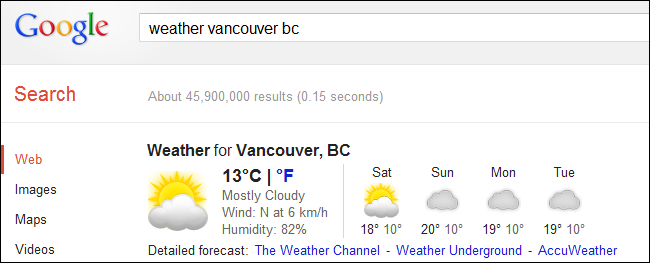The screenshot showcases a Google search result page for "weather in Vancouver, B.C." The top of the page indicates there are approximately 45,900,000 results found in 0.15 seconds. The search options displayed include "Web," "Images," "Maps," and "Videos," with "Web" currently selected, highlighted by a red bar and red text to the left. The remaining options are shown in simple black text beneath it.

To the right of these search options, the current weather information is prominently displayed. The text "weather" is in bold, followed by the word "for" in regular font, then "Vancouver, B.C." in bold again. The temperature reads 13 degrees Celsius, with an option to select Fahrenheit as well. 

A weather graphic illustrates the current conditions: a sun shining partially behind a white, fluffy cloud, indicating mostly cloudy weather with a wind speed of 6 kilometers per hour coming from the north. The humidity level is marked at 82%.

A four-day forecast appears below the current weather details, covering Saturday through Tuesday. The forecast provides high and low temperatures for each day:
- Saturday: 18°C high and 10°C low
- Sunday: 20°C high and 10°C low
- Monday: 19°C high and 10°C low
- Tuesday: 19°C high and 10°C low

This weather information is sourced from The Weather Channel, Weather Underground, and AccuWeather, all enclosed in a small, black, one-pixel frame.